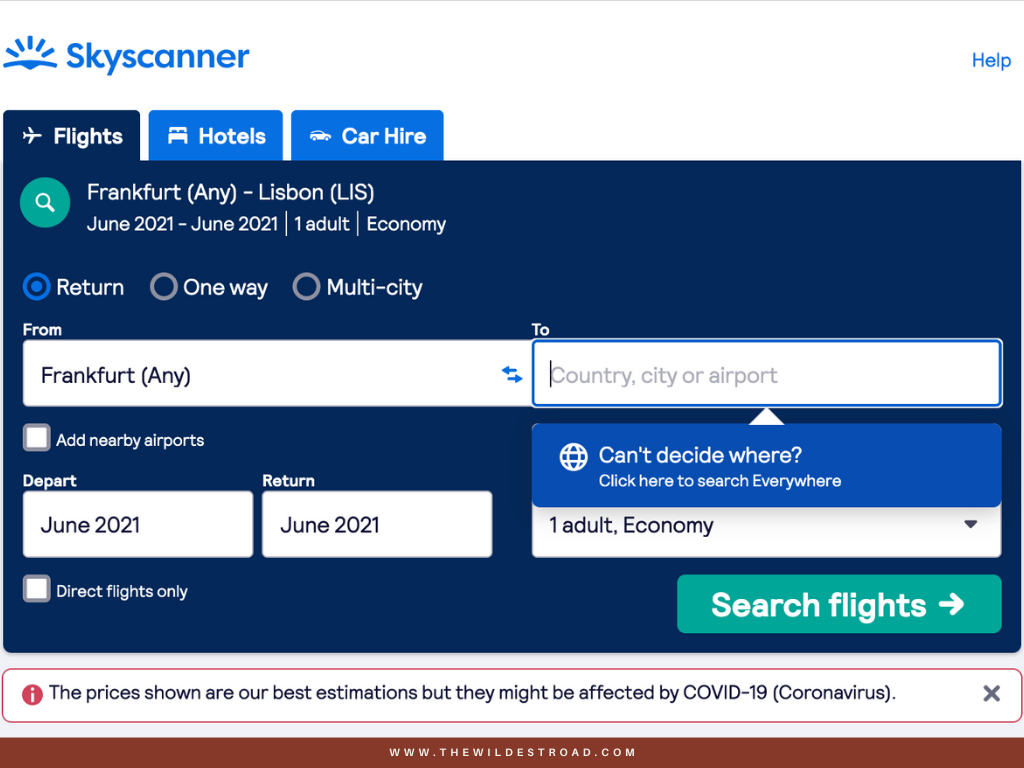In this image of the Sky Scanner webpage, the top left corner features the Sky Scanner logo with both the text and icon in blue. To the top right, there is a "Help" button written in blue on a white background. Below the webpage's name, on the top left, there are navigation tabs for "Flight," "Hotel," and "Car Hire." These tabs are styled with blue backgrounds and white text, except the "Flight" tab, which is highlighted in dark blue.

The main content area of the page has a dark blue background with white and black text. Immediately below the "Flight" tab, it states "Frankfurt, Lisbon, Lisbon, June 2021 to June 2021, one adult, economy." Below this, there are three selectable options: "Return," "One Way," and "Multi-City." The "Return" option is selected, indicating a round-trip search from Frankfurt.

Further details prompt users with "Can't decide where? Click here to search everywhere," accompanied by a checkbox option labeled "Add Nearby Airport." The travel dates are set with "Depart, June 2021" and "Return, June 2021." There's another checkbox for "Direct Flights Only."

On the right side of the form, a green "Search Flights" button awaits action. Beneath this button, a notification in black text on a white background warns, "These prices shown are our best estimations but they might be affected by COVID-19," with the text outlined in red to signify its importance.

At the bottom of the page, the text "www.dwildwestroad.com" is written in white against a brown background accent.